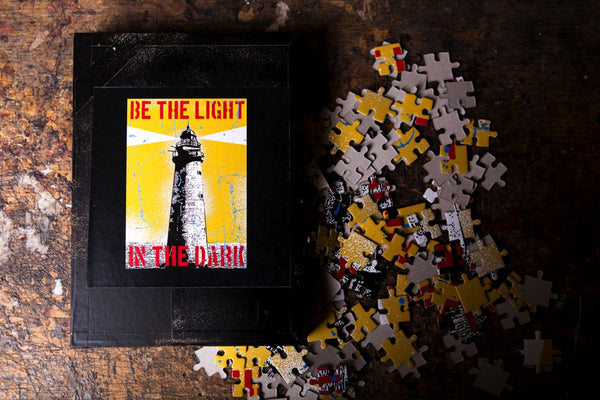A picture of a puzzle set displayed on a dark, worn wooden table with black cuts and scratches. On the left side of the image, the finished puzzle is depicted on a black box with a yellow label, displaying a faded black and white ink drawing of a lighthouse emitting beams of light against a yellow background. The words "Be the light in the dark" are prominently written in red text. The right side of the image shows a dense pile of scattered puzzle pieces, some upside down, featuring the puzzle's colors of red, yellow, white, and black. The table on which the pieces land appears dirty and heavily textured, resembling an old cutting board. The scene encapsulates the comparison between the completed puzzle image and the mixed, unassembled pieces.